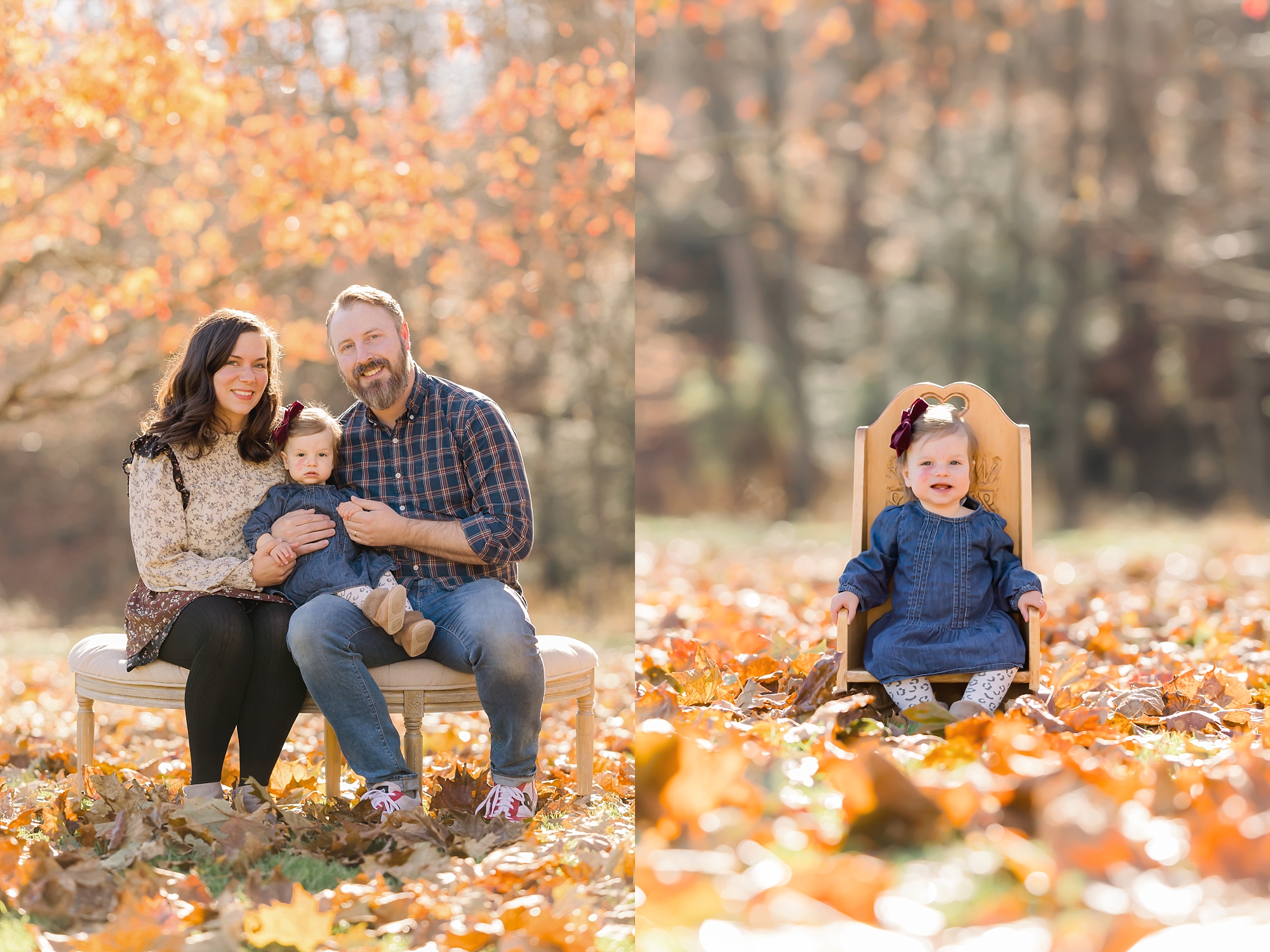This is a wide rectangular image composed of two side-by-side portraits of a family, set against an autumnal backdrop. The left photograph captures the mother and father sitting on a beige fabric bench with their daughter nestled between them. The ground is carpeted with multicolored fall leaves, and the distant background features blurry, orange-hued trees. The mother, with long brown hair, is dressed in a white and red flowered dress paired with black tights. The father sports a blue and red plaid button-up shirt, blue jeans, and tennis shoes. Their daughter, who appears to be a toddler, is wearing a denim dress, spotted leggings, tan boots, and a red bow in her hair. The parents are smiling warmly, though their daughter looks less enthusiastic.

In the right photograph, the setting remains the same with the fall leaves and orange trees in the background. However, this portrait focuses solely on the daughter, who is now sitting on a golden throne-like chair. Unlike the previous image, she is smiling, adding a contrasting mood to this second portrait. This dual composition emphasizes the family’s bond and the autumnal atmosphere in which the photos were taken.